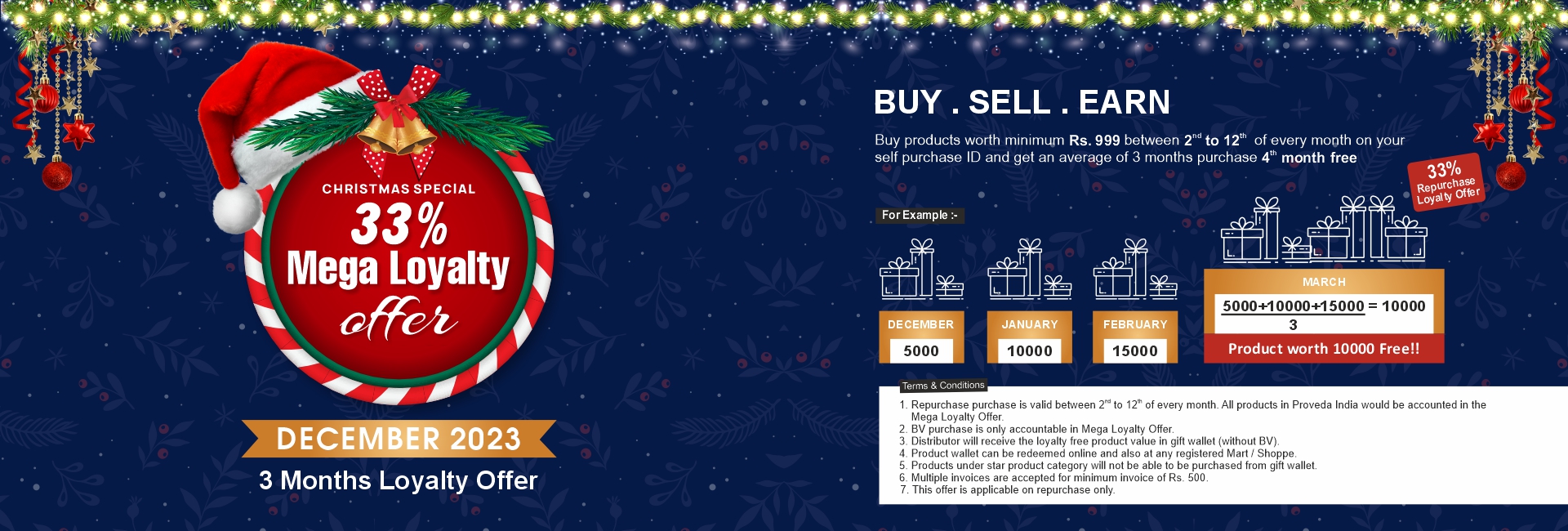Here is the clean and detailed caption for the image described:

---

The promotional material appears to be either a webpage banner or a physical letter centered around a Christmas-themed special offer. On the left side, there is an ornament adorned with a Santa hat and bells, featuring the text "Christmas Special 33%" prominently displayed. Beneath this, it states "December 2023, 3 Months Loyalty Offer".

On the right side of the banner, the text "Buy, Sell, Earn" is highlighted, followed by smaller text explaining the details of the offer: "Purchase products worth a minimum of 9.99 rubies between 2 to 12 inches in height each month on your self-purchase ID and receive an average month's purchase value free over the three-month period."

Below this detailed offer description, examples are provided to illustrate how the benefits work. At the bottom of the banner, there is a small section with terms and conditions, consisting of seven points that outline the specifics of the promotion.

---

This caption provides a structured and comprehensive description of the image.